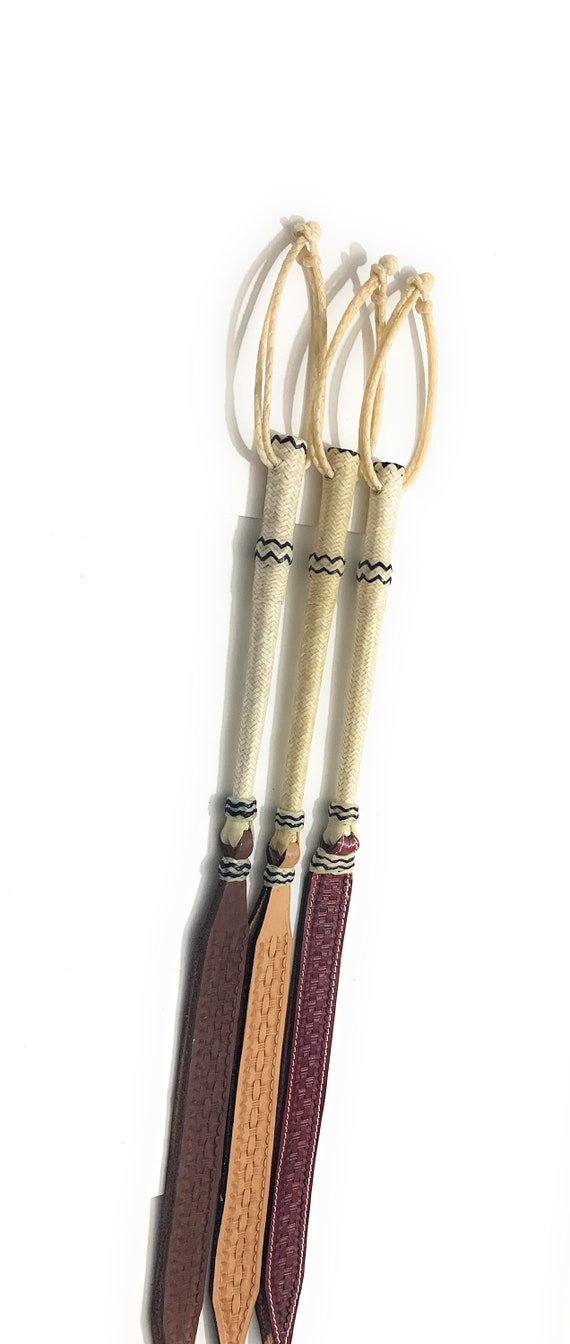The photograph features three vertically aligned, elongated objects set against a white background, with lighting from the right casting subtle shadows to the left. These objects are similar in shape but vary in color: one is dark brown, another is tan, and the third is maroon. Each object has a round, off-white handle adorned with a looped, yellowish cord tied at the top where a small knot is visible; these loops suggest a grip for holding. The handles are detailed with a couple of squiggly black or dark gray lines near their upper sections. Extending from these handles are long, woven sticks that are off-white and enhanced with thread in some sections. At the bottom of each stick, there are longer strips that might be either leather or textured fabric, adding to their distinct appearance. These strips are consistent in their placement but differ in color, matching the main hues of the objects.